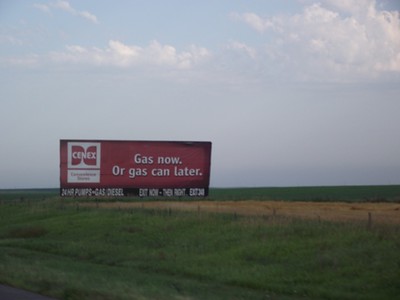A pristine blue sky with wispy clouds graces this picturesque scene dominated by a large billboard on the right side of an open field. The sky, occupying about two-thirds of the image, features light blue hues with scattered, delicate clouds—denser on the left and wispier on the right. Below stretches a verdant landscape, with lush green grass interspersed with patches of exposed brown soil in the foreground, hinting at a rural setting.

The focal point, a vibrant red billboard positioned closer to the right, commands attention. The bold red background frames a prominent Cenex logo, which resembles two intertwined D shapes—or perhaps an 'N'—within a white box. Beneath this logo, another white box contains additional text, though it is not clearly legible. The lower section of the billboard is stark black, featuring white lettering that reads: "Gas now or gas can later. Exit now, third right," and includes an exit number. A phone number is faintly visible on the right side of the billboard.

The combination of the tranquil landscape and the striking billboard creates a visually balanced image, though the simplicity of the setting gives it a somewhat unremarkable, everyday feel.